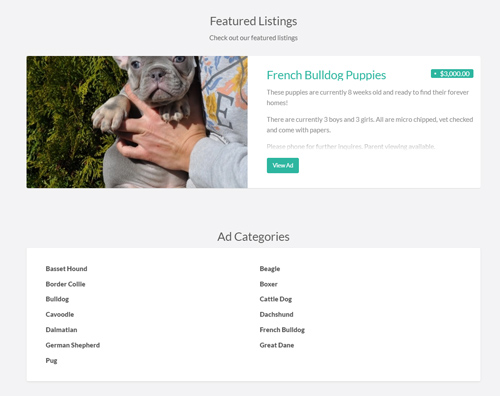This image appears to be a mock-up, possibly a real website template or a conceptual design for a pet breeder's site. At the top center, in bold text, it reads "Feature Listings." Below this header is a photograph of a woman wearing a gray sweatshirt adorned with a heart graphic, holding a young, gray French Bulldog (Frenchie). The Frenchie has a cute face and light blue velvet-like fur, with its paws and belly partially visible. Behind the woman, there is a background of lush greenery, likely ferns or shrubs. 

To the right of the image, in a greenish-teal font, it says "French Bulldog Puppies, $3,000." This section elaborates that the puppies are currently eight weeks old and ready to find their forever homes. It details that there are three males and three females available, all of whom are microchipped, vet-checked, and come with the necessary papers. Below this text, a thin cut-off line separates the details from a rectangular button, also in teal, labeled "View Ad." A gray line extends under the entire image, demarcating it from the subsequent sections.

At the bottom of the page, in a very minimalist white background, there's a list under the heading "Add Categories," featuring various dog breeds: Basset Hound, Border Collie, Bulldog, Cavoodle, Dalmatian, German Shepherd, Pug, Beagle, Boxer, Cattle Dog, Doxen, French Bulldog, and Great Dane. The simplicity and lack of further detail on the page suggest that this design might be a template rather than an actual, fully developed breeder’s website.